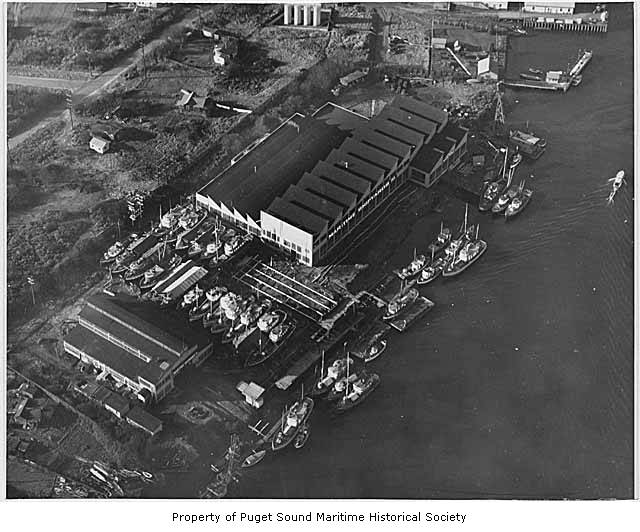This black and white aerial photograph, labeled as property of the Puget Sound Maritime Historical Society, captures an extensive shipyard or port area. Central to the image is a large, long rectangular industrial building with many angled rooftops, and an attached smaller rectangle structure on its left side. Surrounding this building are numerous boats, meticulously lined up both on land and docked in the water adjacent to the structure. In the right portion of the image, a large body of water can be seen with a tiny boat creating visible ripples as it moves through the serene, flat surface. To the far left, roads lead into the area, cutting through a grassy dune-like region where there are a few small structures dotted around.